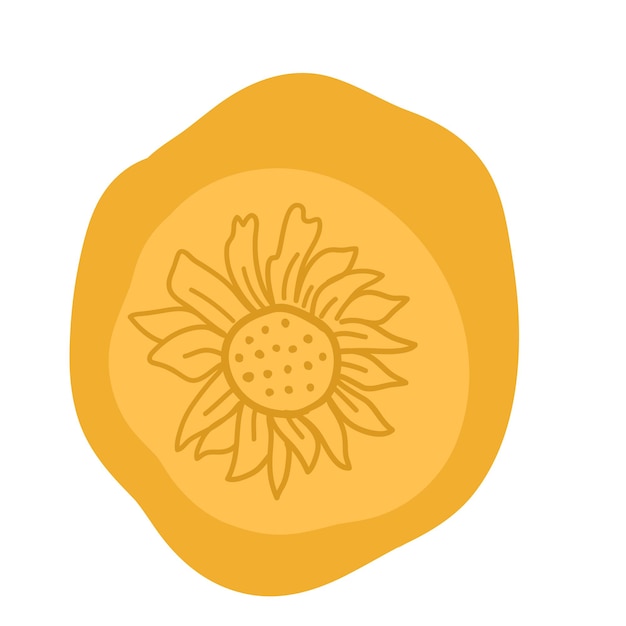This image depicts a digital illustration with a stark white background, focusing on a stylized sunflower. Central to the composition is a roughly oval, warm golden-yellow shape with wavy, irregular edges, giving it a lumpy appearance. Within this outer shape lies a slightly more circular, lighter golden-yellow form. At the heart of this inner shape is a simple line drawing of a sunflower, executed in the same warm golden hue as the outer contour. 

The sunflower features approximately 18-20 asymmetrical, elongated petals of various shapes and sizes, each detailed with a vein down the middle. The flower's center contains a cluster of around 16-20 dots representing seeds. The overall design bears a resemblance to clip art or vector graphics and combines elements that hint at both artistic representation and potentially fossilized imagery. The minimalist nature of the image, with its contrasting yellow tones and simple lines, evokes a sense of modern digital art.